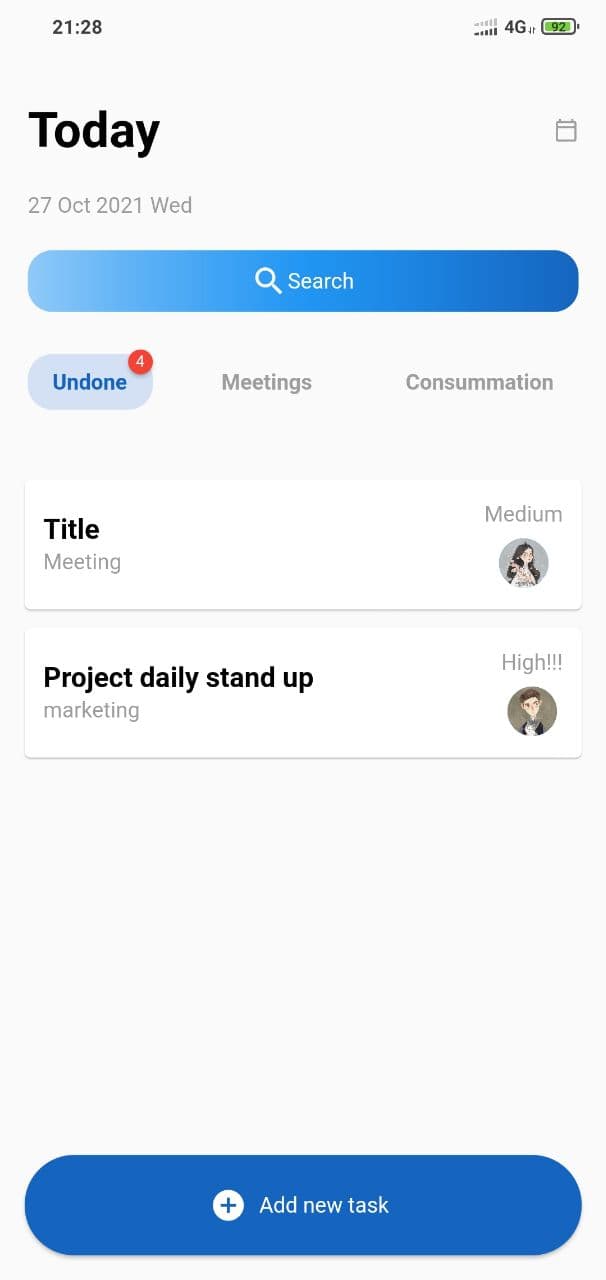In this image, we see the front view of a smartphone against a plain white background. The screen displays a 4G network status and the time "21:28" in grey print at the top. Below this, in large bold black letters, the word "Today" is prominently displayed. Beneath in smaller grey letters, the date is noted as "27th October 2021, Wednesday."

On the right side of the screen, there is a small rectangular box. Adjacent to this is a gradient blue search button, fading from light blue to dark blue, with the word "Search" written in white. 

Further down, a light blue section with darker blue text highlights "Undone," which seems to be the selected category. A red circle with the number "4" next to it signifies the count of tasks or notifications. Below this, the words "Meetings" and "Consummation" are listed.

The "Undone" section is followed by titles of specific tasks or events. First, it says "Title" with "Meeting" written underneath. Additionally, there is a "Medium" priority label, and a small circular thumbnail displaying a girl's photo indicating an assignee. The task "Project Daily Stand-Up" is labeled under "Marketing." To the right, a circular thumbnail shows a picture of a guy with a greeting "Hi!!!" beside it.

At the bottom of the screen, there is a blue button with a white circle containing a blue plus sign, captioned "Add New Task."